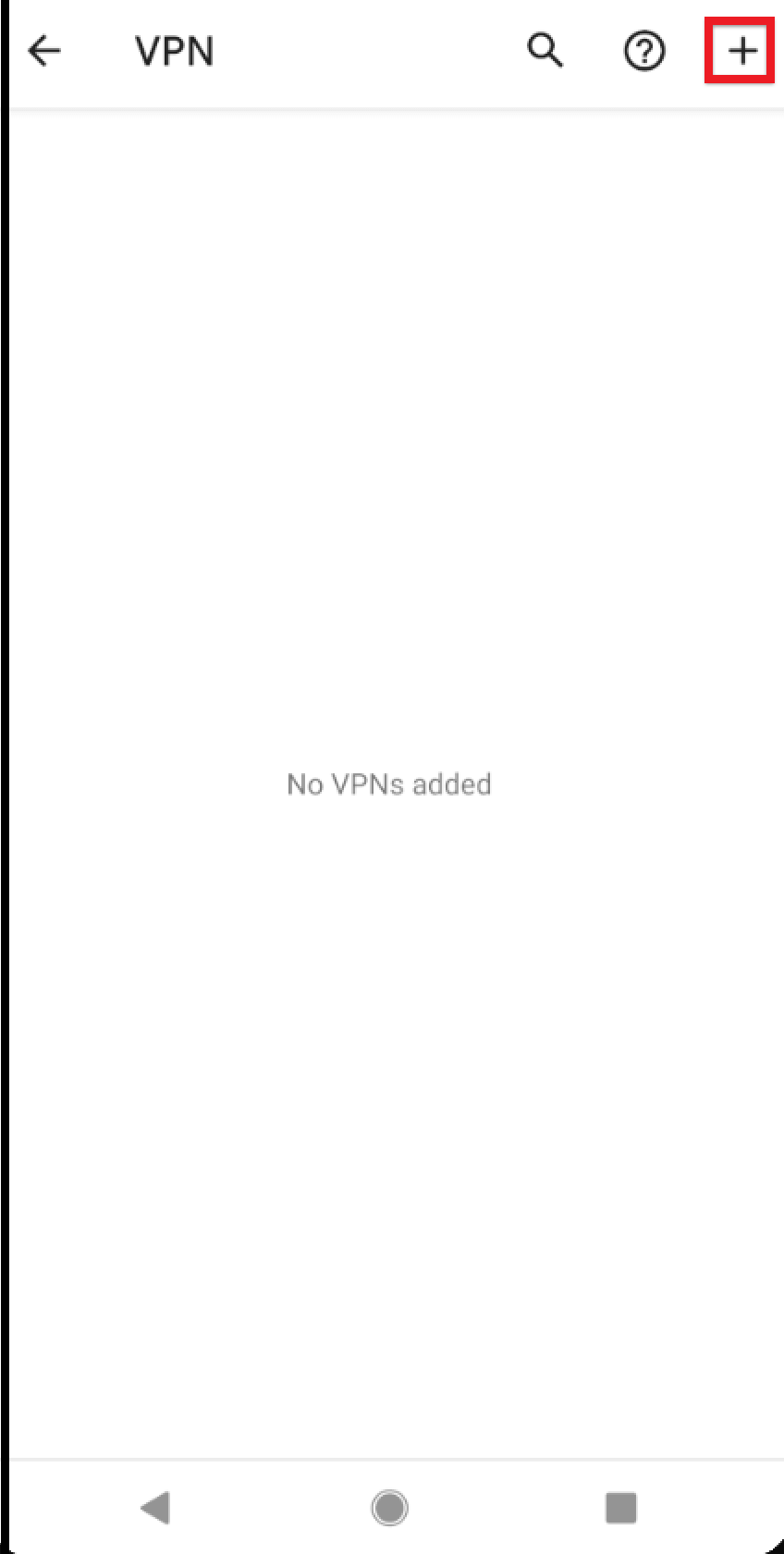The image depicts a smartphone screen displaying a VPN settings page. The screen has a predominantly white background with several UI elements. At the top, a left-pointing black arrow labeled "VPN" is visible, indicating that this is the VPN settings section. To the right of the "VPN" label, there are three icons: a search icon, a question mark icon inside a circle, and a red box with a black square in the center, possibly representing a button to add a new VPN.

In the middle of the screen, in gray text, it says "No VPNs added," confirming that no VPN configurations are present on the device. A thin, black line runs vertically along the top left edge but stops before reaching the bottom. The right side of the screen also has minor visual details but remains mostly white towards the bottom.

At the bottom of the screen, typical navigation icons of an Android device are visible: a left-pointing arrow (back icon), a circle (home icon), and a square (recent apps icon). These elements indicate that the screenshot was taken on an Android device, and the user is in the process of managing VPNs on their phone.

The red box with a black square in the top right corner is likely a button to add a new VPN, suggesting interactivity for the user to input new VPN details. The overall color scheme is minimalist, featuring mainly white, black, gray, and the small red element for the add VPN button.

It seems that the bottom part of the image has been cropped or cut off, perhaps unintentionally, when it was captured or uploaded.